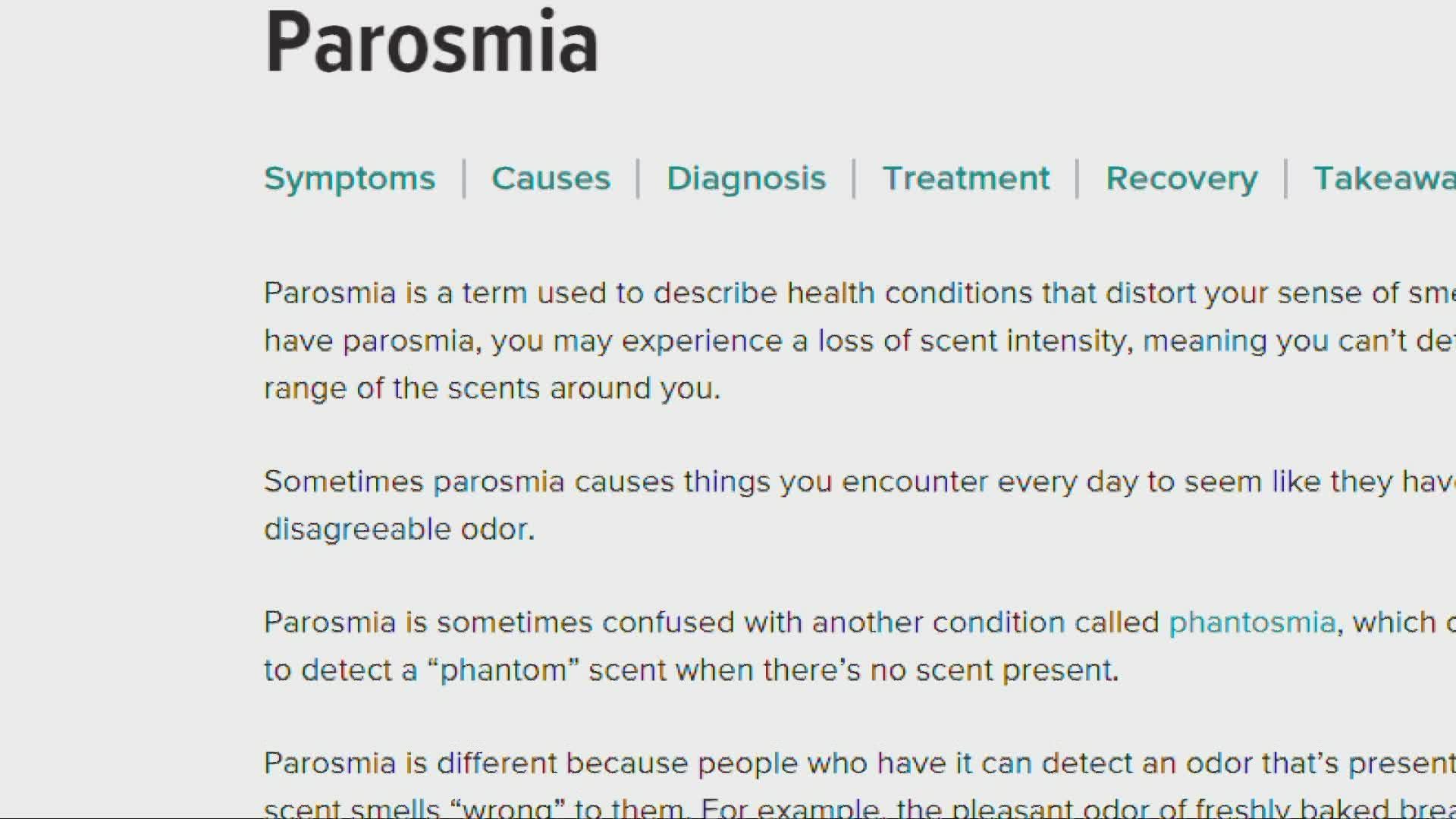This partial screenshot captures an informative webpage about Parosmia. The image is incomplete, with parts of the right-hand side and bottom sections of the page missing, indicating a need to scroll both vertically and horizontally to view the entire content. The topmost and largest text, written in black against a light gray background, unmistakably displays the title: "Parosmia."

Beneath this title, there are several greenish-colored, clickable text links that presumably navigate to different sections of the webpage. These links are labeled as follows: "Symptoms," "Causes," "Diagnosis," "Treatment," "Recovery," and "Takeaways."

Further down, the visible part of the screenshot shows four paragraphs, although some lines are truncated. These paragraphs appear to provide an overview of Parosmia and offer insights into identifying the condition.